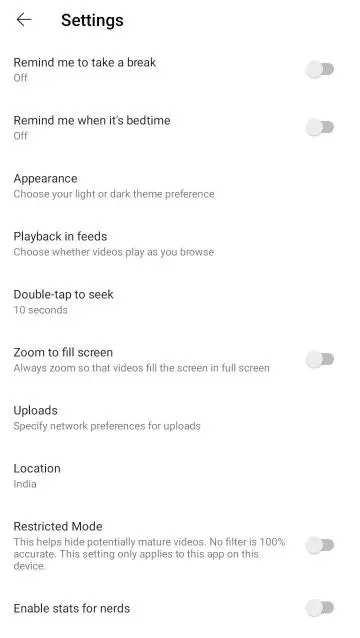In the top left corner of the image, there is a small arrow pointing to the left, next to the word "Settings" in black text. Below this, the text reads "Remind me to take a break," with the word "Off" in small letters underneath. To the right of this text, there is a toggle switch positioned to the left, indicating it is off.

Further down, the text reads "Remind me when it's bedtime," followed by the word "Off" underneath. A small toggle switch to the right of this text is also placed to the left, indicating it is off. 

Below these settings, in bolder black text, is the word "Appearance." Underneath this, it states "Choose your light or dark theme preference."

Continuing down, the text "Playback and feeds" appears, followed by "Choose whether videos play as you browse." Below this, another option, "Double tap to seek," is set to "10 seconds." 

Next, there is an option titled "Zoom to fill screen," which reads "Always zoom so that videos fit the screen in full screen" underneath.

Below that, the text "Uploads" appears, describing this section as specifying network preferences for uploads.

Further down, the section titled "Location" has "India" written underneath it.

Continuing, the "Restricted mode" option states "This helps hide potentially mature videos. No filter is 100% accurate. This setting only applies to this app on this device."

Finally, at the bottom, the last option is "Enable stats for nerds," which is toggled off, shown by a left-positioned toggle switch.